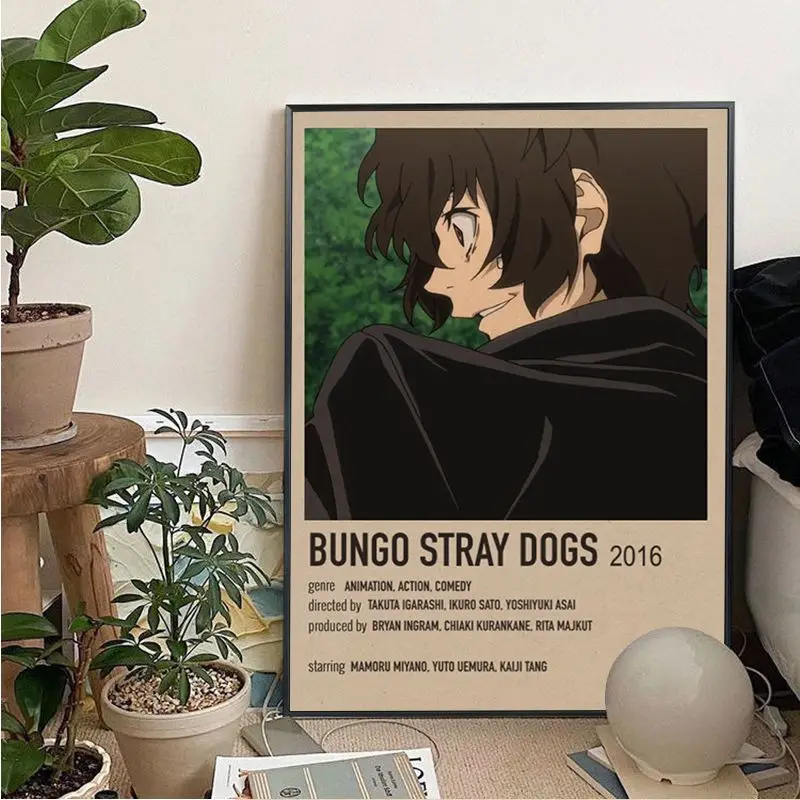The image is a detailed indoor color close-up of a framed movie poster for "Bungo Stray Dogs," a Japanese animated film released in 2016. The poster, prominently featuring an anime character, occupies the top two-thirds of the frame. The character, depicted in a profile view, has shaggy brown hair, a grimacing expression, and is partially obscured by a dark cape or cloak. The lower part of the poster includes important details, such as the film's title, genre (animation, action, comedy), and production credits. Surrounding the poster on the cluttered floor are potted plants—two placed directly on the floor and one sitting on a small wooden stool, along with scattered books and papers. A distinctive round lamp is visible in the right corner of the image. The white wall in the background contrasts with the lively, detailed scene in the foreground.